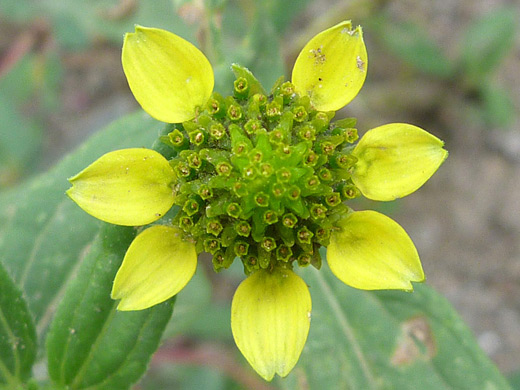In this close-up photograph taken in daylight, the focal point is an intriguing plant that defies easy classification as a flower. At the center, a round formation hosts a cluster of tiny green growths, resembling sprouting buds. Surrounding this central cluster are approximately seven teardrop-shaped petals, which are predominantly yellow with subtle green tips. Each petal, although mostly intact, displays slight damage, possibly from insects, evidenced by small missing sections and white spots. Flanking this composition are large, almond-shaped leaves in a rich green hue. The background remains muted and blurred, accentuating the plant's detailed features, while the lower left corner distinctly captures a single, vibrant green leaf.